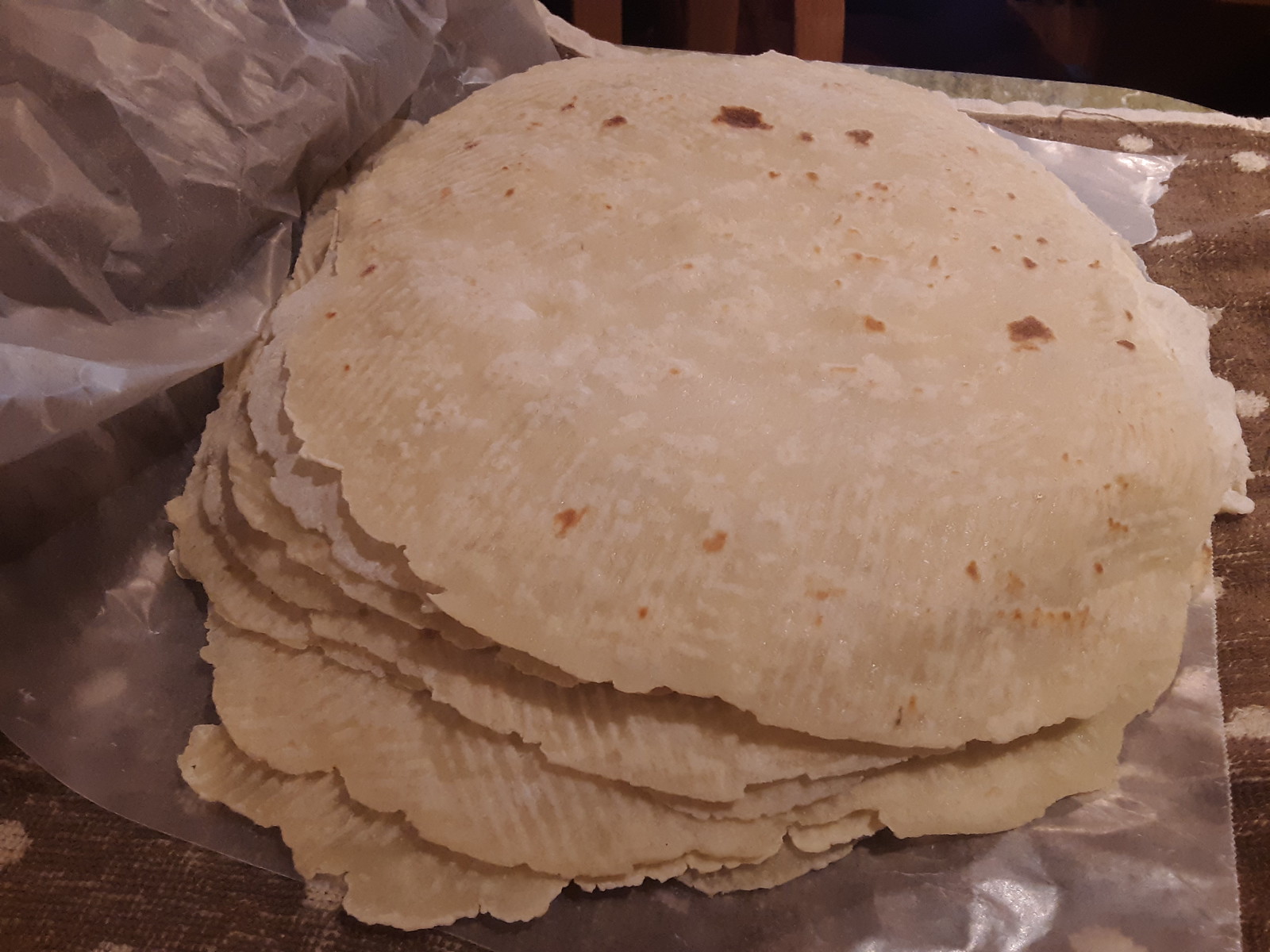In this close-up photograph taken with a personal camera, we see a stack of several homemade tortillas, roughly a dozen or more, laid out on a thin plastic or wax paper. The wax paper, which appears crinkled and uneven on the right side, forms the base for these tortillas and is laid atop a brown tablecloth with subtle tannish circle dots. The tortillas are a classic off-white color with noticeable brown spots and jagged edges, indicative of their handmade nature. Their circular forms are almost perfect but slightly irregular, emphasizing their homemade charm. The top tortilla exhibits typical cooking marks and striations, suggesting they are freshly prepared and ready to eat. In the background, three wooden poles are faintly visible, adding a rustic feel to the setting. The overall composition and detailed textures hint at a moment of culinary creation, inviting the viewer to appreciate the nuances of these freshly made tortillas.